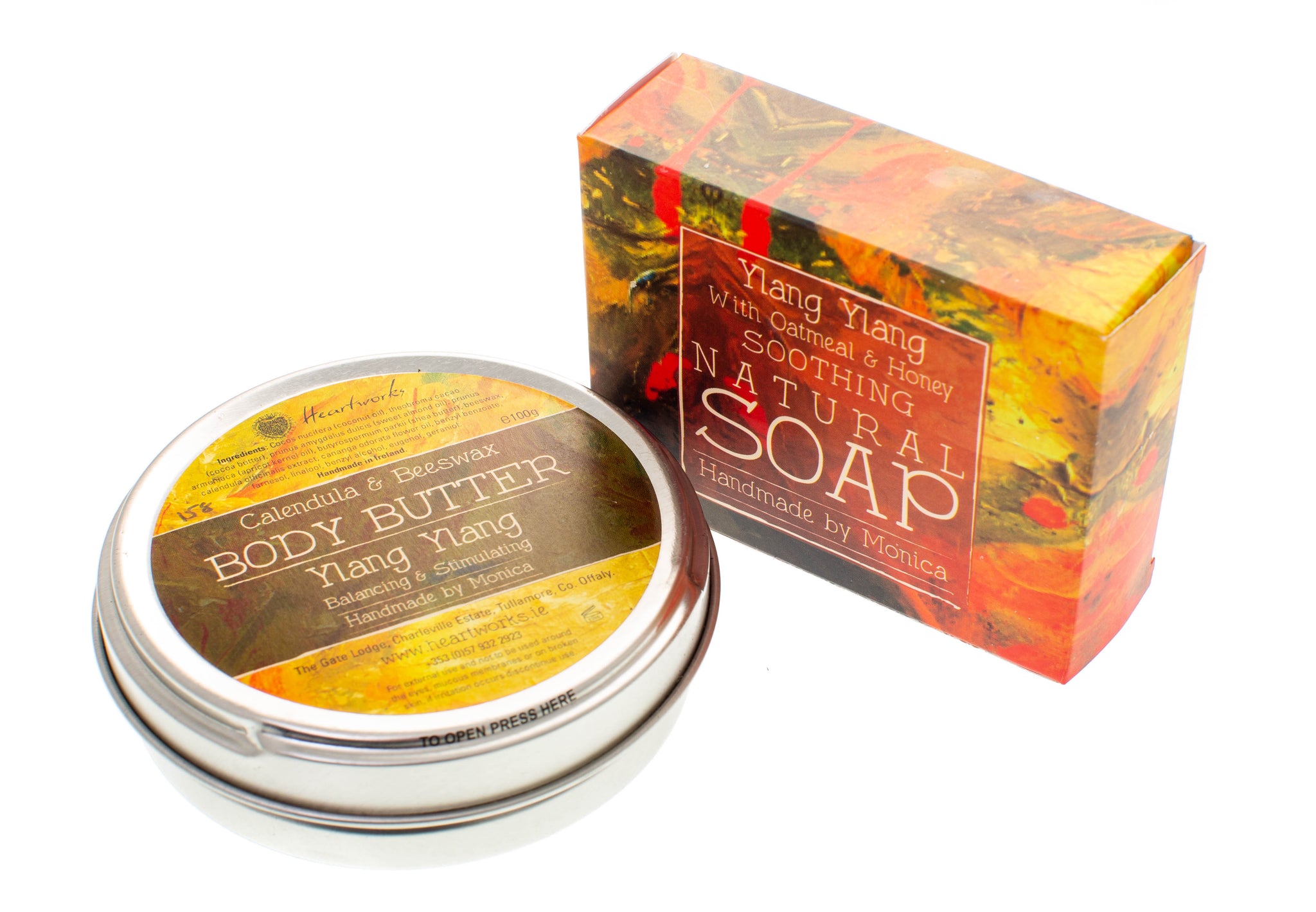This image, a color photograph in landscape orientation, features two bath products against a stark white background, emphasizing their details. On the left, there's a shallow, round silver tin of body butter. This tin has a sticker on the lid with a yellow background and a large brown horizontal bar in the center. The text on the sticker reads "Calendula and Beeswax Body Butter, Ylang Ylang, Balancing and Stimulating, Handmade by Monica." Some additional text is present on the yellow part of the sticker but is unreadable from the distance. 

To the right of the tin is a box containing an individual bar of soap. The box, standing on its edge at an angle, features an abstract floral design in shades of yellow, orange, red, and green. At the center of the box is an orange square with white text that reads "Ylang Ylang with Oatmeal and Honey, Soothing Natural Soap, Handmade by Monica." The photograph represents the products realistically, allowing them to visually pop against the clean background, typical of product photography in a representational style.